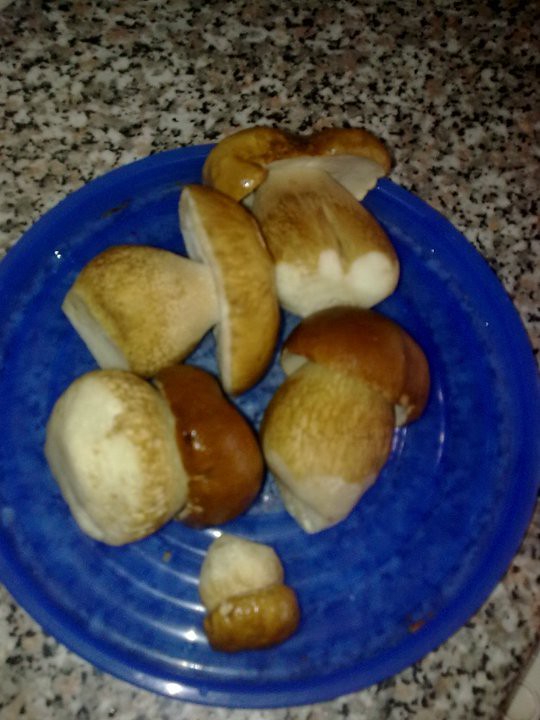In the center of this amateur photograph, a group of five mushrooms is arranged on a translucent blue Tupperware lid, which sits atop a speckled black-and-white granite countertop. Four larger mushrooms form a square, with their caps displaying shades of light to dark brown: two with lighter caps at the top and two with darker caps on the bottom. The smallest mushroom, positioned at the center bottom of the square, has a medium brown cap and stands out because of its size. The largest mushroom, located in the top left, presents its cap upwards, visibly displaying its underside. The top right mushroom also has its cap facing up, while the bottom-left mushroom, with its darker cap and fat stem, pairs closely with the adjacent mushroom on the right. The lid, slightly see-through and blue, prominently contrasts with the textured countertop, grounding the otherwise earthy tones of the mushrooms.